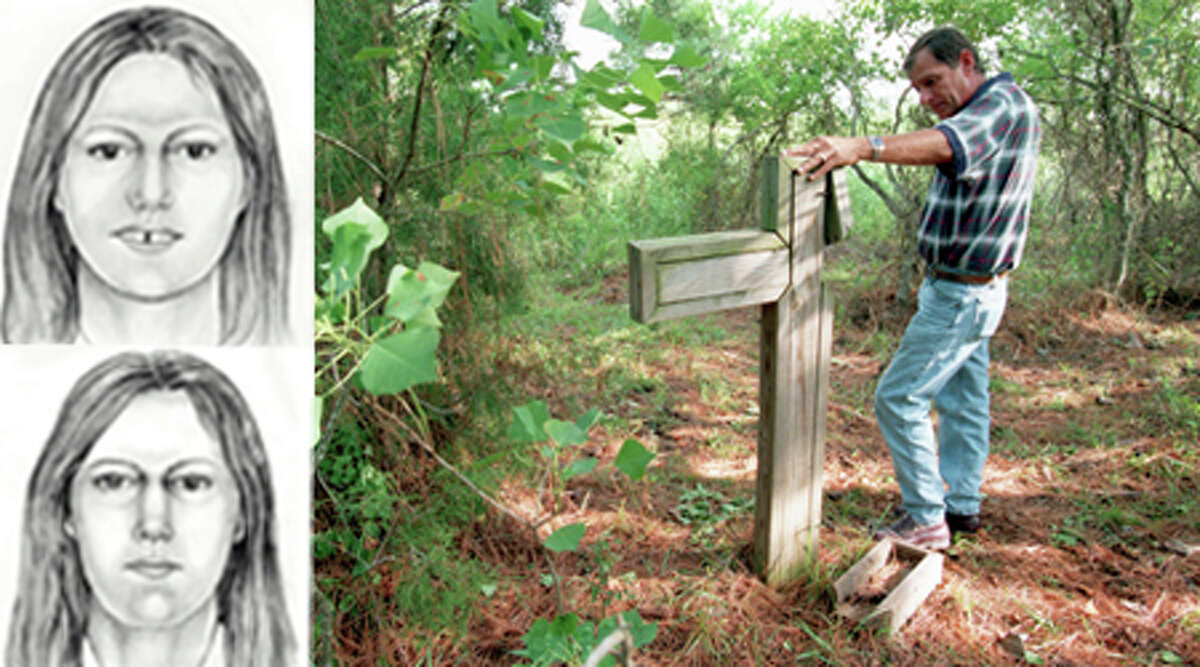The image depicts a solemn scene set in a lush forest, characterized by thin trees with wide green leaves and a ground covered in brownish soil and small tree parts. Central to the image is a man dressed in blue jeans and a multicolored shirt, including shades of blue and green. He stands beside a weathered wooden cross, part of which is broken off and held in his left hand as he gazes downward, seemingly contemplating how to repair it. To the left of the man are two black-and-white sketches of women. The top sketch features a woman with long dark hair and a noticeable smile that reveals a missing front tooth, while the bottom sketch depicts another woman with similar long dark hair but a more elongated face and serious expression. The backdrop of the scene is accentuated by the natural, bright light filtering through the forest canopy, giving a clear and poignant view of this memorial-like setting.